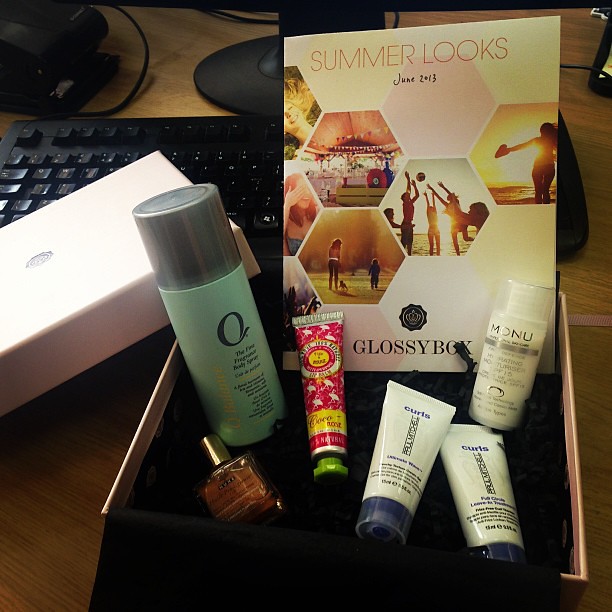A desktop with a woodgrain surface showcases a neatly arranged unboxing of beauty products, complete with a black computer keyboard and monitor in the background. Central to the image is a white gift box with a black liner, prominently displaying various cosmetics. The box cover is leaned against the keyboard, partially obscured by a booklet that reads "Summer Looks, June 2013, Glossy Box." The box contains six distinct beauty items meticulously laid out: a square glass jar with a cap, a brightly colored and flamingo-printed lip balm tube, a perfume bottle with a large "Q" logo, two matching bottles from the brand "Curls" likely indicating shampoo and conditioner, a blue-green tube with a gray cap possibly containing moisturizer or sunscreen, and another dispenser on the right labeled "MONU." The setup suggests an unboxing intended to showcase the variety of cosmetics within this Glossy Box edition.